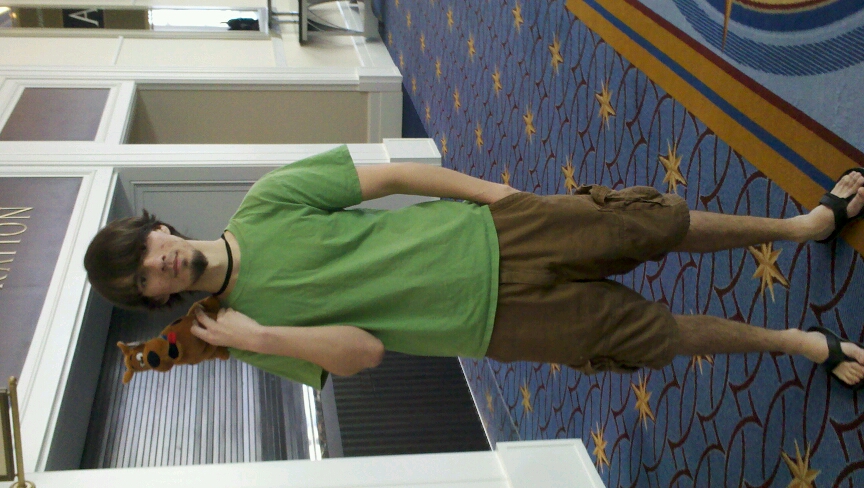A man is dressed up as Shaggy from Scooby-Doo, complete with a small, light brown Scooby-Doo stuffed animal perched on his right shoulder. His attire includes a green t-shirt, khaki cargo shorts that hang low over his knees, and black sandals. He accessorizes with a black necklace and sports a surf-style haircut and a black goatee, further enhancing his resemblance to the character. He stands on a blue carpet adorned with yellow stars and lines, within what appears to be a hotel setting. Behind him, there is a window with shutters and a table, suggesting the possibility of a Comic-Con event. The man gazes directly at the camera, capturing the essence of Shaggy in both appearance and ambiance.